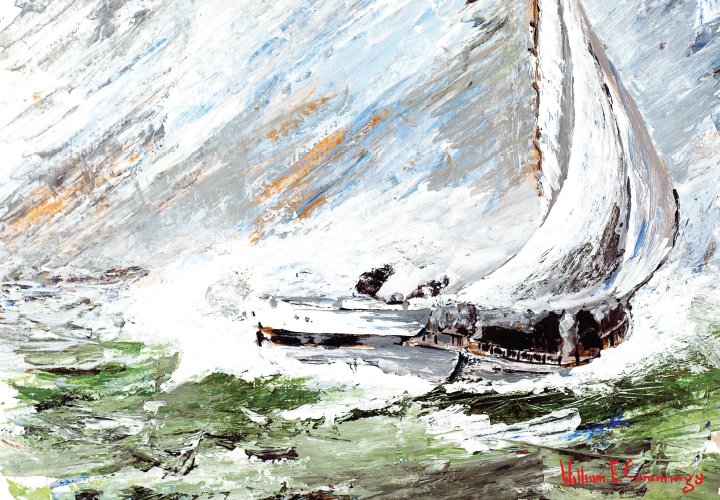This painting is a wide canvas depicting a dramatic maritime scene with a signature in red at the bottom right, reading “William L. Lumming.” The focal point of the artwork is a black sailboat with a white sail, filled with wind, navigating through rough, green waters accented with whitecaps. Despite the turmoil of the sea, the boat appears unoccupied. The background sky is painted with dynamic, fast brush strokes blending white, gray, blue, and bits of orange, reminiscent of a stormy or rainy atmosphere. The style of the painting exhibits a painterly technique, with visible strokes contributing to its somewhat abstract impression.